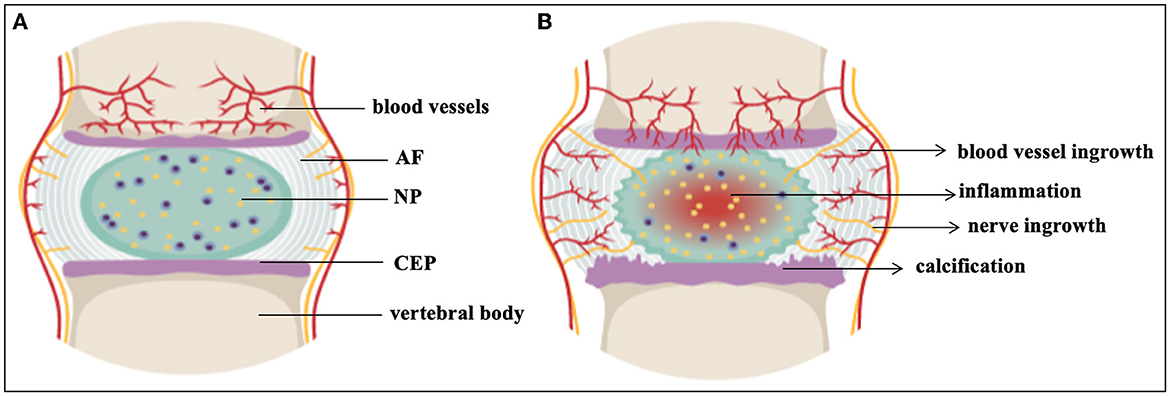This infographic features two rectangular, cartoonish-style medical diagrams labeled A and B, depicting the progression of a disease in a vertebral body, possibly part of the spine. Diagram A shows a healthy state with clear labels for blood vessels, AF, NP, CEP, and vertebral body. The illustration includes a blue circular area with dots, flanked by white regions above and below, and red lines surrounding it. Diagram B contrasts sharply, illustrating the diseased state with labels indicating blood vessel ingrowth, inflammation, nerve ingrowth, and calcification. The overall image has a small black border surrounding the detailed drawings.